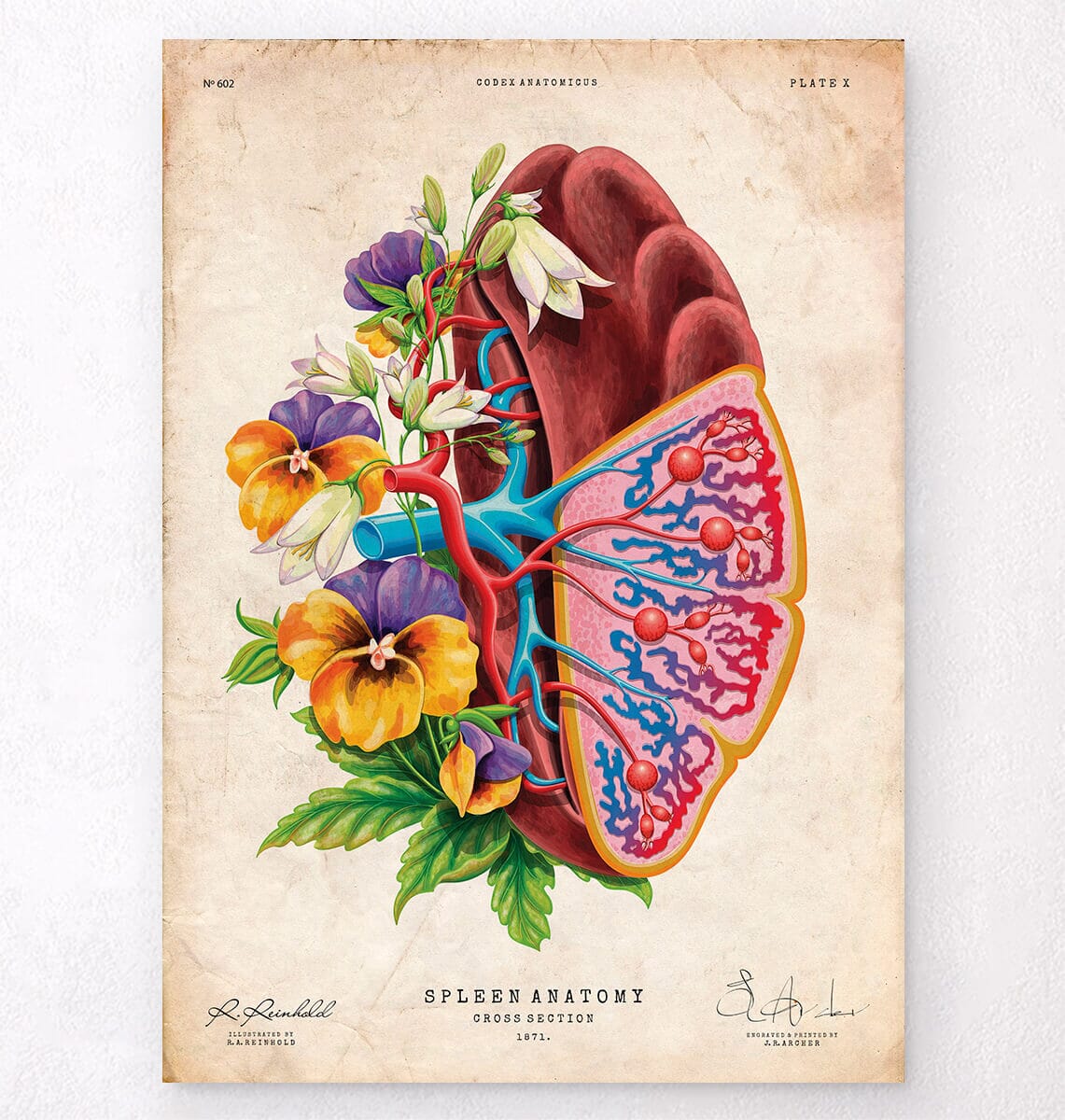The image is a detailed and elaborate illustration of a human spleen's anatomy, set against an old, weathered paper with a white background that appears brown and faded along the edges. At the top, written in small black font, it reads "Number 602" in the top left, "Codex Anatomicus" in the top middle, and "Plate X" in the top right. The artistic work is attributed to R. Reinhold and J.R. Archer, with their signatures located at the bottom left and right, respectively. The central illustration is titled "Spleen Anatomy Cross Section 1871," situated in the bottom middle.

The spleen is depicted in a vertically-oriented position with a reddish-brown exterior. The cross-sectional view reveals an intricate network of blue and red blood vessels. Beyond its anatomical accuracy, the illustration uniquely incorporates an array of vibrant flowers and foliage growing out of the left side of the spleen. These include orange, purple, white, and yellow flowers, some resembling pansies and bell-shaped blooms, accompanied by green leaves and buds. The overall design interlaces scientific precision with artistic embellishments, making it both informative and visually captivating.